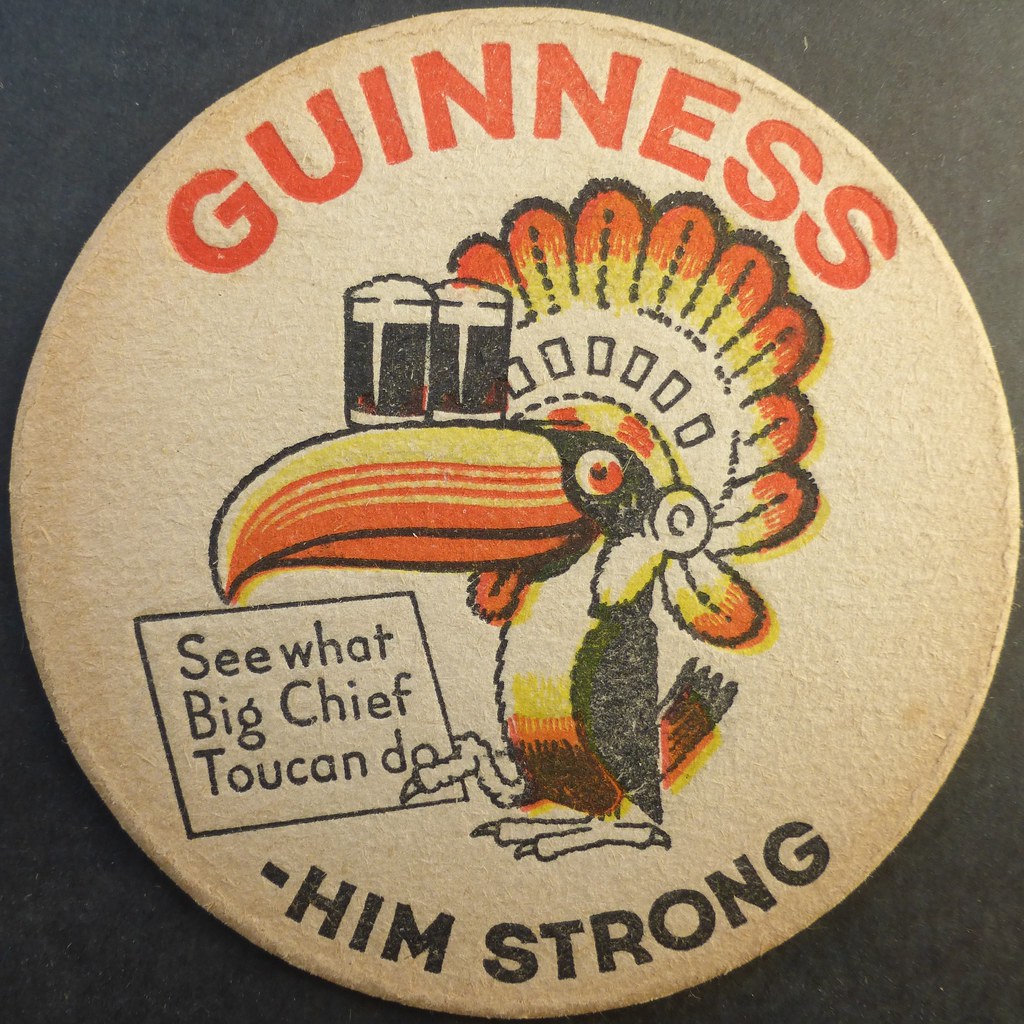The image features a square coaster with a dark gray to black background. Centered prominently is a large off-white circle that reaches the top, bottom, left, and right edges of the coaster, seamlessly touching all four sides. Within this circle, a stylized drawing of a toucan is showcased, facing left. The toucan has a distinctive black head and a long beak that points to the right, colored in vibrant shades of yellow and orange and outlined in black. The bird's body is predominantly white, adorned with accents of yellow and orange.

Adding to the toucan's unique appearance is a headdress resembling an Indian headdress, with feathers colored in orange and yellow. Perched atop the toucan's beak are two glasses filled with a dark liquid topped with a white foamy head, likely representing pints of Guinness. Above the toucan, in large orange letters, the word "Guinness" is prominently displayed. At the bottom of the circle, in bold black letters, it reads "him strong." Additionally, the toucan is holding a card in one of its feet, which bears the message, "see what Big Chief Toucan can do," written in black ink. The detailed and playful design suggests that the item depicted is a coaster, possibly used for promotional purposes.